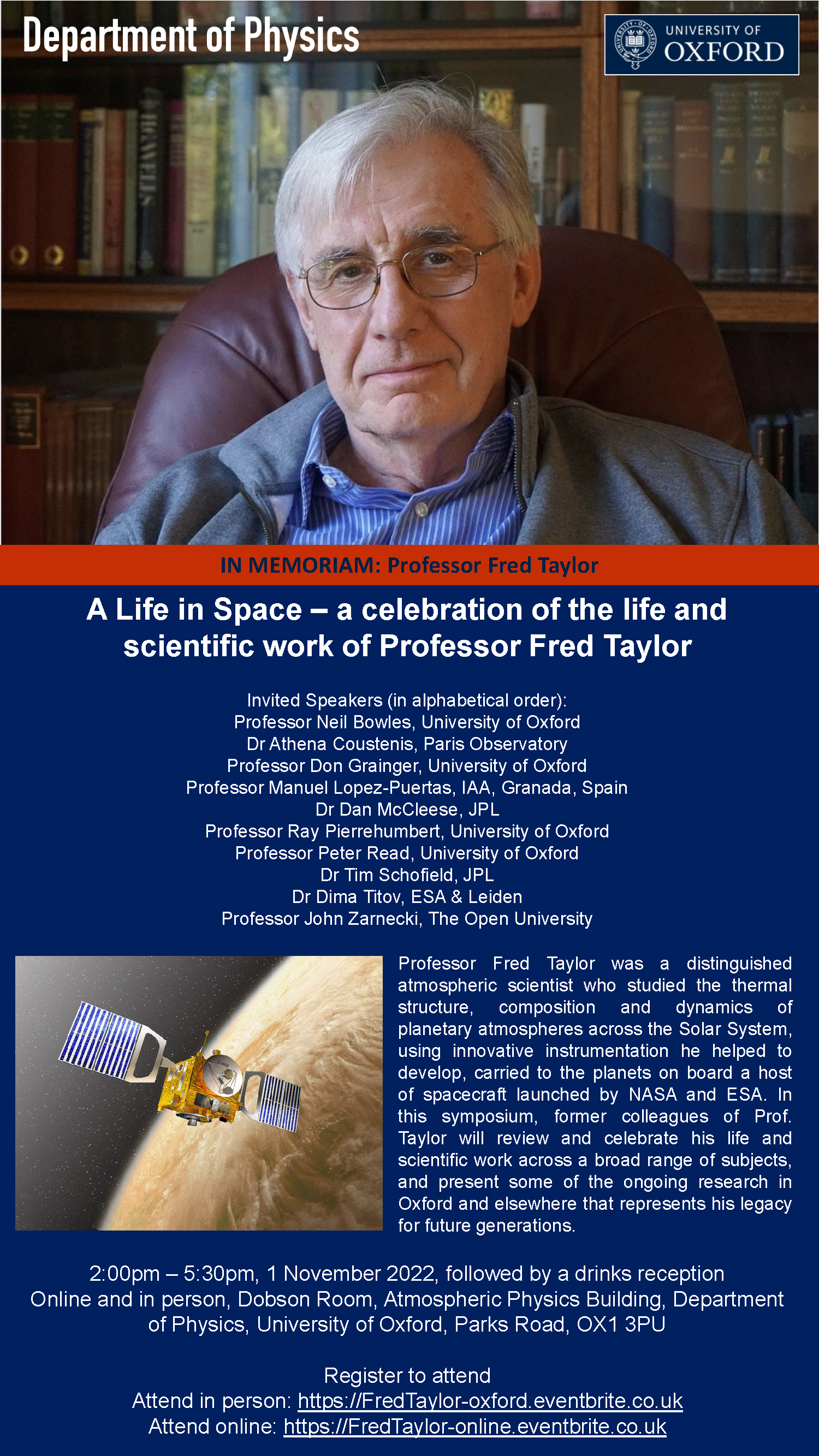The poster from the Department of Physics at the University of Oxford commemorates Professor Fred Taylor. At the top, it features the University of Oxford logo and inscription in a blue rectangle. The central image is a photo of Professor Taylor, an older man with glasses and a tired expression, seated in a leather chair with a bookshelf behind him. A red rectangle caption underneath reads "In Memoriam, Professor Fred Taylor," followed by a large blue section stating "A Life in Space: A Celebration of the Life and Scientific Work of Professor Fred Taylor." Below this, the poster lists invited speakers in alphabetical order: Professor Neil Bowles (University of Oxford), Dr. Athena Kosenis (Paris Observatory), Professor Don Granger (University of Oxford), Professor Manuel Lopez Burgess (IAE, University of Spain), Dr. D.M. McLeese (JPL), Professor Ray Piren-Rutenberg (University of Oxford), Professor Peter Reed (University of Oxford), Dr. Tim Schofield (JPL), Dr. Dima Teotiavi (USA), and Professor John Zarnacki (UP University). The poster highlights Professor Taylor's distinguished contributions as an atmospheric scientist who extensively studied the thermal structure, composition, and dynamics of planetary atmospheres across the solar system. He developed innovative instrumentation for NASA and ESA spacecraft. The symposium will review and celebrate his life and scientific work, featuring presentations on ongoing research connected to his legacy. The event will take place from 2 p.m. to 5:30 p.m. on November 1, 2022, followed by a drinks reception in the Dobson Room, Atmospheric Physics Building, University of Oxford, Parks Road, OX13PU. Registration is available online at HTTPS://fredtaylor-oxford-eventbranch.co.uk for in-person attendance and HTTPS://fredtaylor-online-eventbranch.co.uk for online participation.